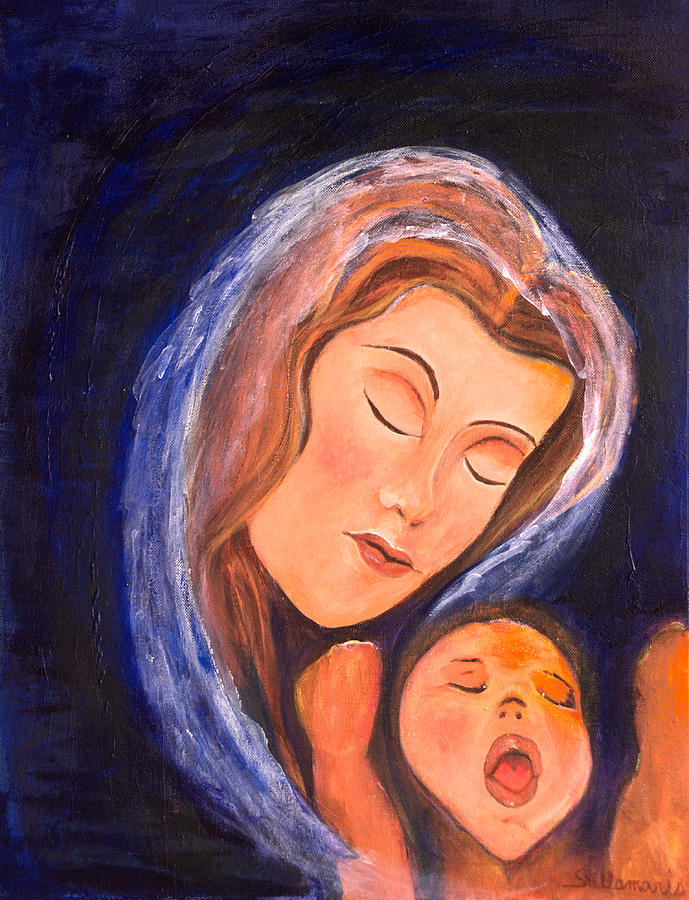This is a painting depicting a tender scene between a mother and her child, set against a swirling, dark navy and black background. The mother, occupying the central part of the image, has long brown hair that transitions to purple and white near the edges. She possesses a light complexion, thin eyebrows, and wears a gentle, almost pursed expression as if preparing to kiss the baby. Her eyes are closed, and her head is tilted downward. A white halo encircles her head, adding a spiritual aura to the piece.

The baby, positioned in the lower right corner of the painting, appears slightly darker in complexion, with short brown hair. Its eyes are closed and its mouth is open wide, possibly crying or yawning, revealing a red tongue. The baby's arms are raised, with one hand close to the mother's chin, and the hands are rendered indistinctly, resembling pallets or out-of-proportion limbs. The mother seems to be soothing the baby.

The artist’s signature, which looks like "Stellamaris," is located in the bottom right corner. The overall effect of the painting is tender yet disquieting, enhanced by the disproportionate features and the expressive, albeit unsettling, portrayal of the child.